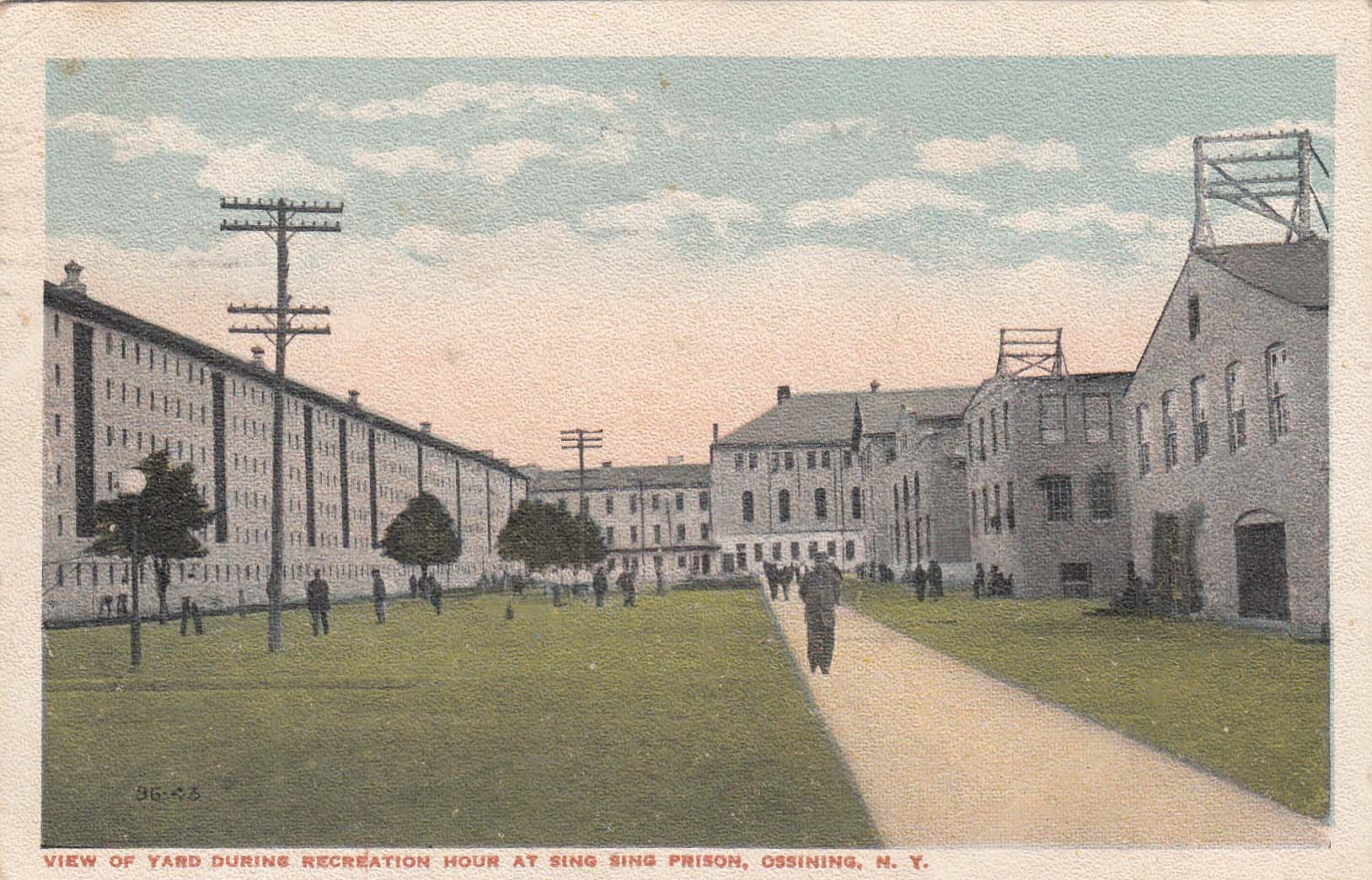This image, seemingly an old, colorized, and grainy postcard, provides a detailed view of the Sing Sing Prison yard in Ossining, New York, during recreation hour. The scene is dominated by gray, nondescript buildings, an eight-story structure on the left and two-story buildings on the right, which enclose the courtyard. The sky is blue and partially covered in clouds, indicating daylight. A wide, gray path cuts through the center of the courtyard, flanked by patches of grass and a few scattered trees. Visible along this path, a solitary figure walks towards the foreground. The yard is sparsely populated with inmates; some are congregated on the field to the left, possibly exercising. The image also features several electricity poles within the yard. A red caption below the image reads, "View of Yard during Recreation Hour at Sing Sing Prison, Ossining, New York."